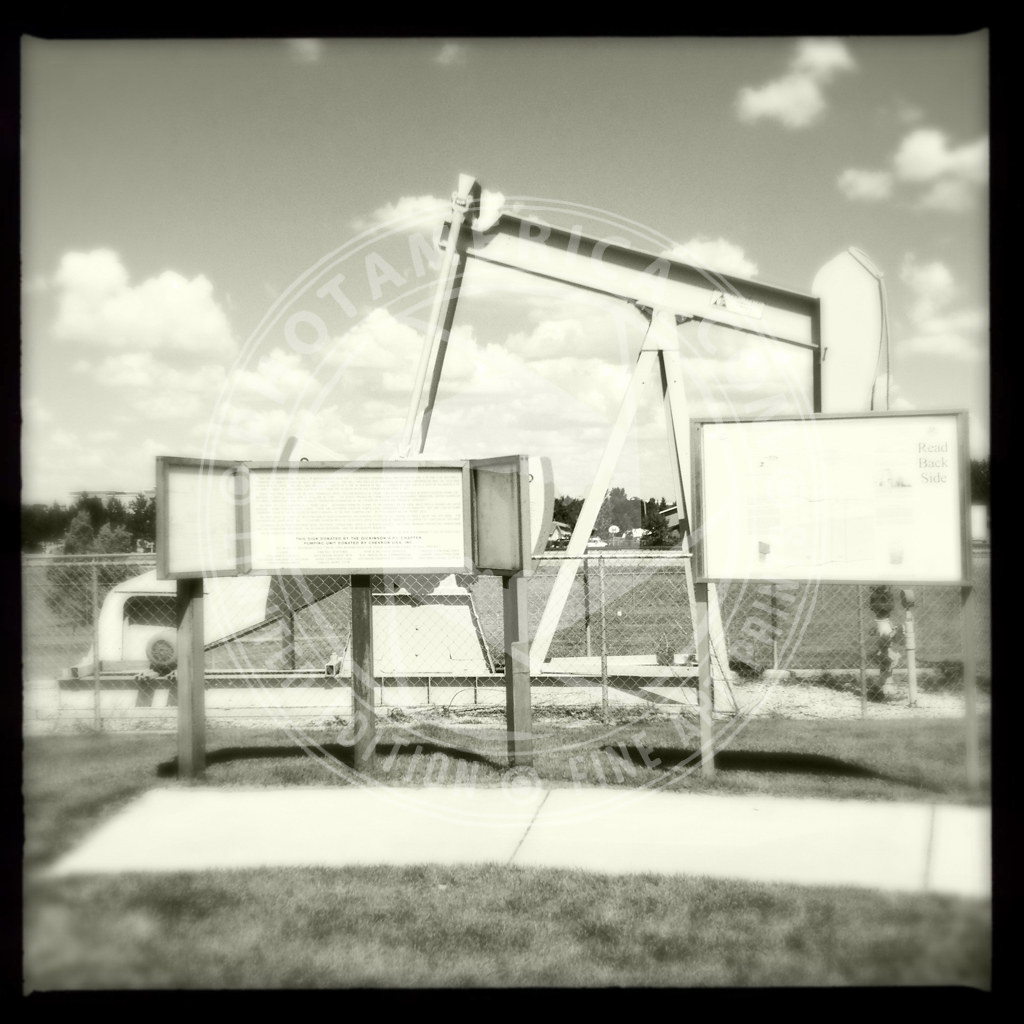This black-and-white photo captures an outdoor scene centered around an oil pump jack, partially visible and set at an angle. The foreground features a small, narrow sidewalk bordered by grass, leading up to several signs mounted on wooden posts. On the left, there is a sign composed of three wooden posts holding a large central rectangle flanked by two smaller squares. These signs have light-colored backgrounds with dark, indiscernible text. Another sign on the right, framed in a rectangular shape, bears a clear message in its upper right corner stating "read back side." In the middle ground, a chain link fence separates the viewer from the pump jack and a surrounding dirt area where the grass does not grow. Behind the oil pump jack, trees dot the landscape, and expansive sky with fluffy white clouds suggests a clear, beautiful day. The image is framed by a narrow, black border and also features a faint, unreadable watermark.